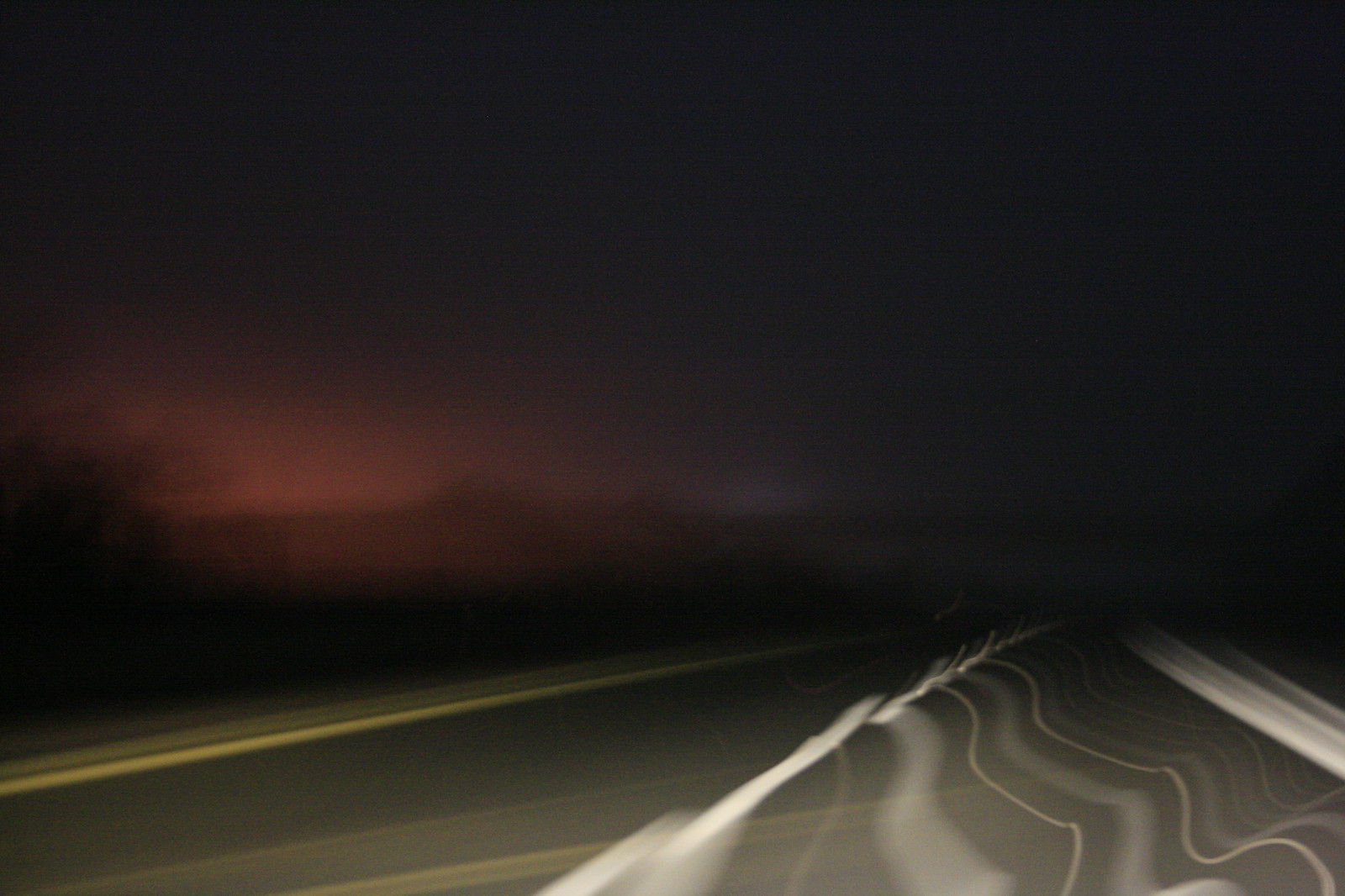This nighttime photograph captures a dark, deserted road. The top third of the image is nearly pitch black, while a mysterious red glow emanates from the left side, halfway up the image, possibly hinting at a distant sunset or sunrise. The scene features two asphalt lanes receding into the dark distance. The shot is taken from the perspective of a vehicle traveling in the right lane, on what appears to be a single carriageway. A central dividing white line runs parallel to a white line on the right side of the lane and a yellow line on the left side of the opposite lane. The lines are blurred and reflect light, possibly due to the movement of the camera or insufficient lighting. The road ahead is only visible for about twenty yards, with no other vehicles in sight, emphasizing the solitude and darkness of the scene.